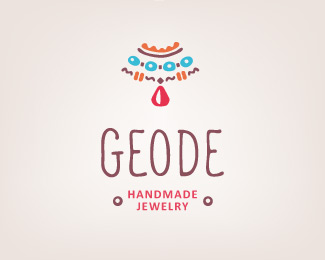The image features a rectangular, light grey frame showcasing a logo or stylized illustration at the top, which appears to represent a piece of handmade jewelry. The design consists of a chain of four teal ovals, each with a white circle in the center and black dots linking them together. Above the oval chain is a red squiggly chain, while below it is a black squiggly chain, from which hangs a red, diamond-shaped pendant resembling a ruby. Directly beneath this design, in large, dark brown letters, is the word "GEODE". Below "GEODE", in smaller red uppercase letters bordered by two brown dots on each side, is the phrase "HANDMADE JEWELRY". This entire composition is set against a cream-colored, textured background, creating an advertisement-like appearance for a jewelry company.